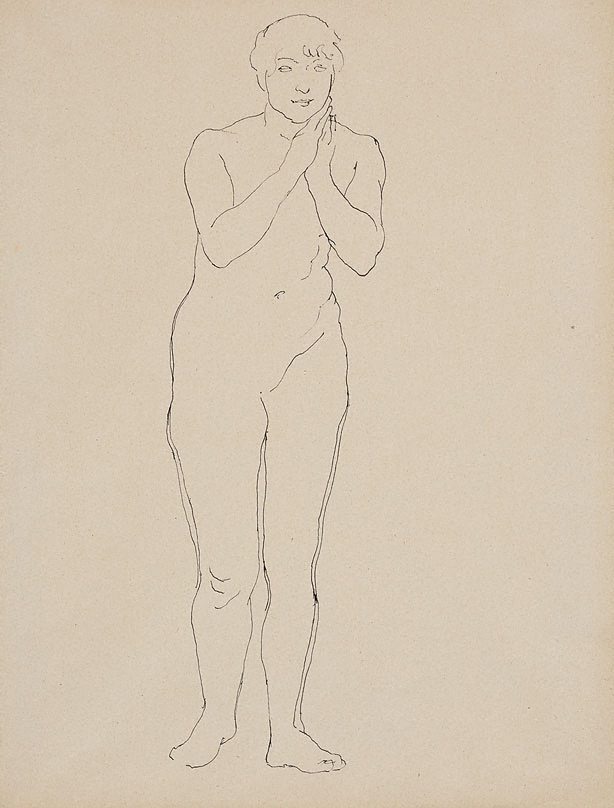This artwork is a simple and rudimentary line sketch of a full-figured human form, likely nude, against a light tan or beige background. The figure appears nude, yet the lack of detail and absence of genitalia leaves the gender somewhat ambiguous, though features like slightly rounded belly, masculine shoulders, and thick thighs suggest a male body. Their short hair is styled, and they stand with their right leg slightly behind the left, hands clasped together near the left side of their neck or under their chin. There are minimal details, with the image defined primarily by simple brown or black lines. Notable features include the belly button and subtle indications of stomach muscles. The figure looks directly outward with a calm expression, possibly a small smile, creating an approachable and somewhat serene mood in the piece.